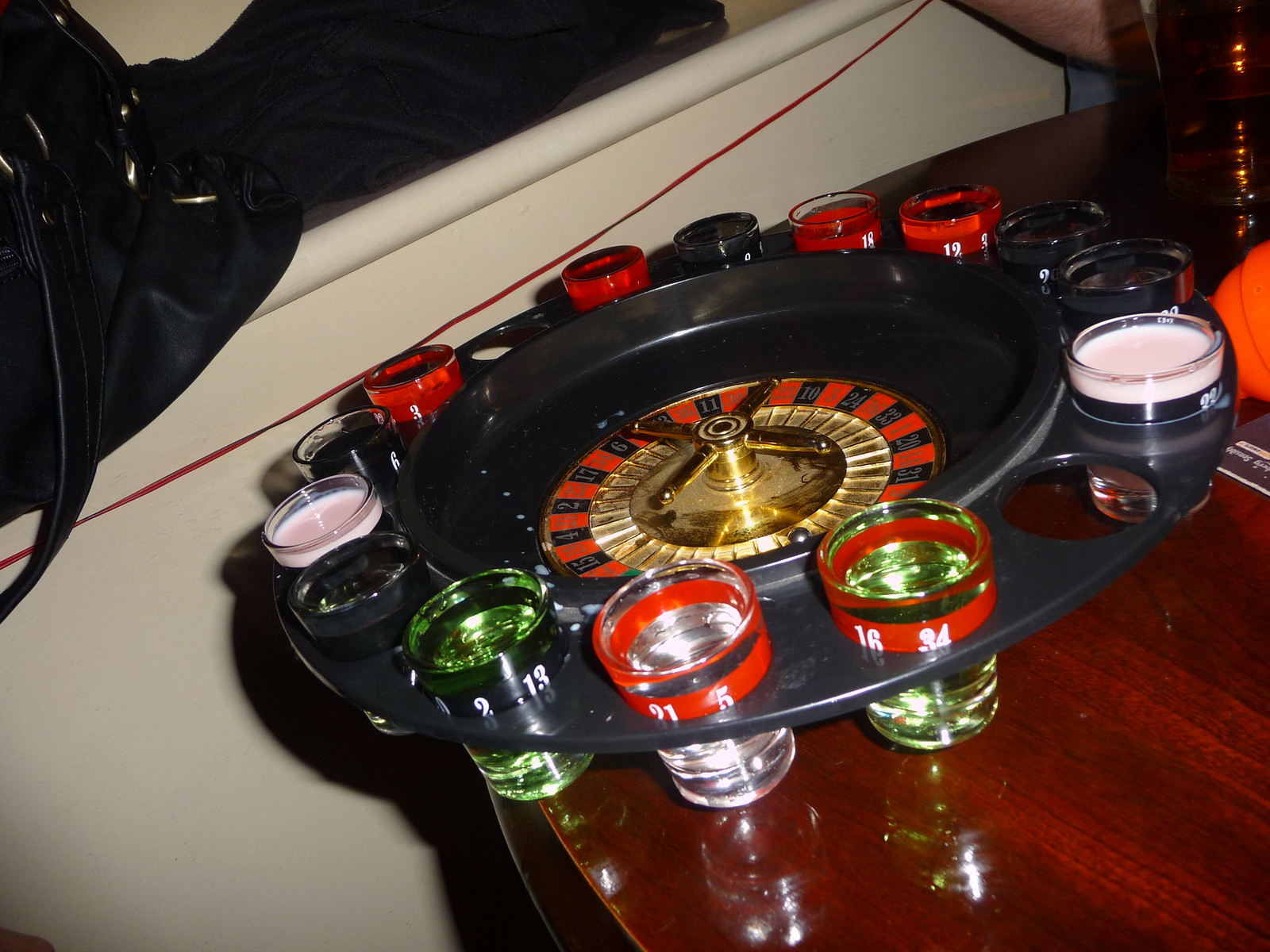The image depicts what appears to be a lively poker night setting, featuring a polished mahogany table with just its edge visible in the shot. Centered on the table is a miniature roulette wheel, encased within a glossy black circular plate. This plate features multiple holes around its periphery, each containing a shot glass. The shot glasses are adorned with blue bands at the top and red bands with numbers, and they contain either beer or clear liquid. The interior of the roulette wheel is golden, displaying the iconic alternating red and black numbered spaces. 

Further in the background, a beige object – possibly a couch – is visible, and a black object, perhaps a purse with a strap, hangs down near the edge of the white surface. A red string lies below the top of a nearby chair, adding another hint of color to the scene. An orange object is noticeable along the top edge of the table’s right side, contributing to the detailed ambiance of this cozy, game-night tableau.